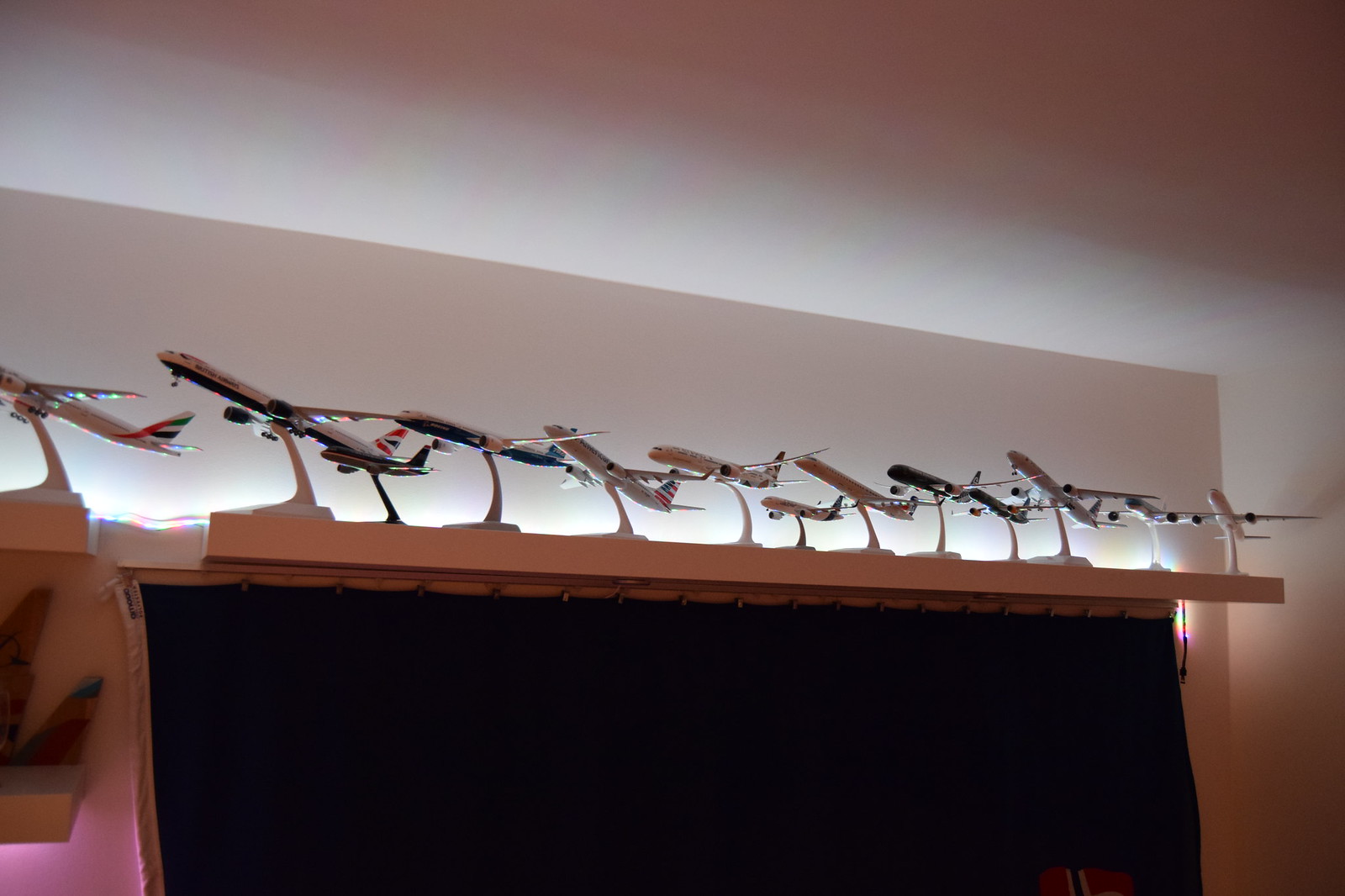This detailed photograph, taken from a somewhat low angle, showcases a collection of 13 model passenger airplanes positioned on a long shelf placed approximately a foot and a half below a white ceiling. The shelf, made of a pale-colored material, extends above a window dressed with a dark, closed blue curtain. The airplanes are mounted on white, round bases with angled stands, causing them to tilt upwards as if they are taking off. They represent various major airline carriers, with most models being primarily white, featuring different airline tail markings, though the specific airlines are not identifiable due to the distance.

The scene is illuminated by a light strip draped across the top of the shelf, casting a bright light on the models. Additionally, ambient lighting in different colors, including red, green, and purple, provides a vibrant backdrop. Part of the light strip hangs beside the curtain, illuminating a nearby wall fixture, identified by some as an abstract artwork. To the left side of the image, a small portion of another shelf with a single model airplane is visible, adding to the depth of the room. The lower back corner of the image includes a pink fluffy object, enhancing the colorful ambiance. Overall, the photograph captures the intricate display and lighting of the model airplanes in a well-organized and detailed manner against a white wall and ceiling background.